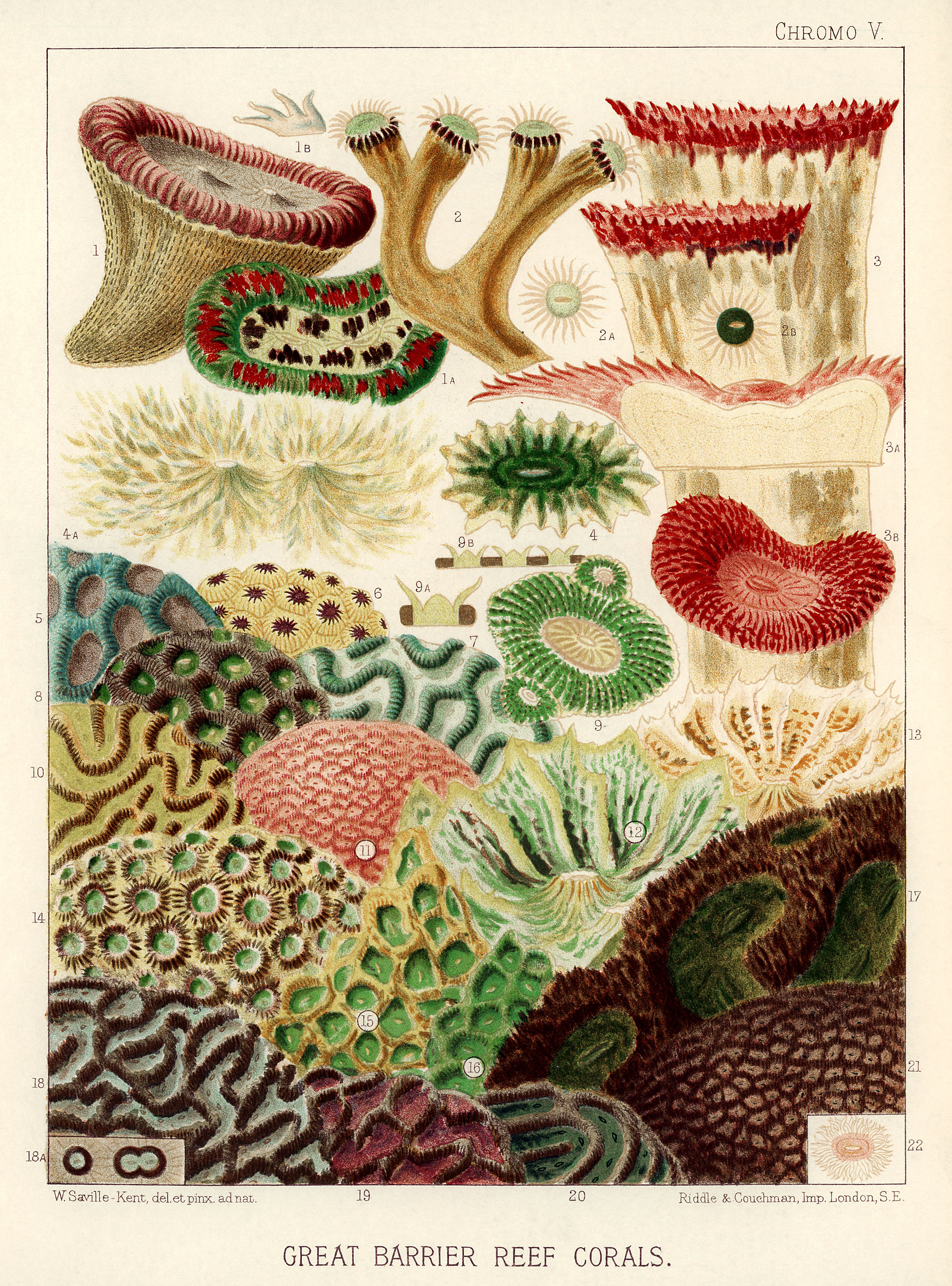This image features a detailed illustration of various coral species from the Great Barrier Reef, depicted on light brown-colored paper. The corals are illustrated in an array of vibrant colors, including coral red, brown, green, wine red, deep red, cream, yellow, and orange. The diverse shapes of the corals, including round forms and others resembling mushrooms, highlight the rich variety of natural organisms found in the reef. Each coral is marked with numbers, suggesting that there is a corresponding legend or key that is not included in the image. At the top right corner, the text "Chromo V." is written, while the bottom middle prominently features the title "Great Barrier Reef Corals."